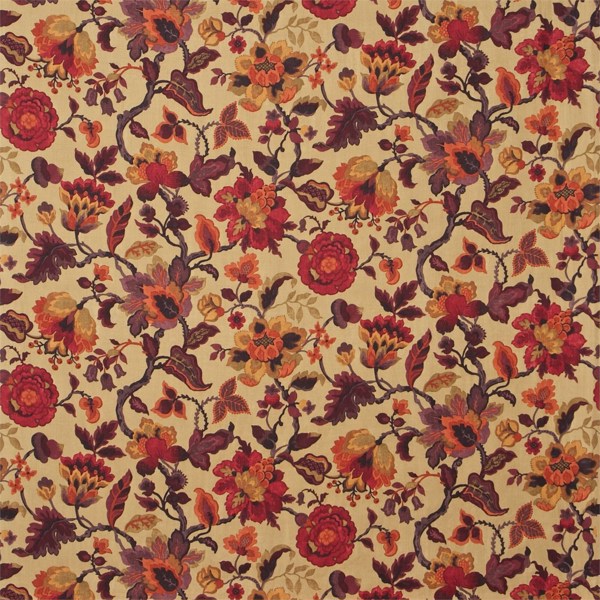This image depicts a detailed, repetitive pattern that evokes the feel of autumn. The background is a light tan or yellowish hue, covered entirely with an intricate floral design. The flowers vary in color, including deep reds, oranges, yellows, and some with purplish tones and red centers. Brown stems and vines intertwine among the blossoms, creating a cohesive, organic aesthetic. Leaves present in the pattern are predominantly brown and orange, further enhancing the autumnal theme. The artwork, whether it be fabric or wallpaper, exhibits a warm, fall-inspired palette with an overall yellow tint, possibly due to lighting conditions during photography.